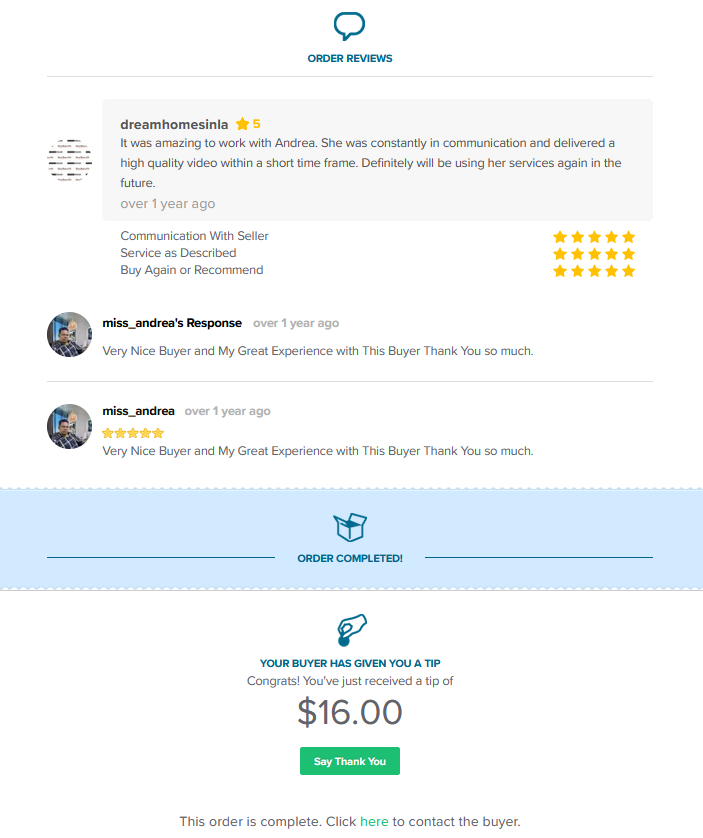**Detailed Caption:**

The image displays an order review summary from a platform where users leave feedback for services received. The highlighted review, titled "Dream Homes Mania," features a prominent five-star rating and praises an individual named Andrea for her exceptional service. The reviewer commends Andrea's counseling, communication, and the swift delivery of a high-quality video. They express their intent to use her services again in the future. This review, dated over a year ago, includes detailed ratings: a perfect five out of five for communicating with the seller, service as described, willingness to buy again, and recommendation.

Andrea responded to the review over a year ago, expressing gratitude: "Very nice buyer and great experience with this buyer. Thanks so much." Notably, this response is repeated, indicating a duplicate entry.

Below this review section, a notification indicates the order has been completed. There is a visual of an open box marked with "ORDER COMPLETED" in all caps, surrounded by a perforated blue line, suggesting it can be cut out. 

An emoji resembling a coin being inserted hints at a monetary tip from the buyer. The notification reads, "Your buyer has given you a tip. Congrats! Receive $16." This section includes a clickable "Say Thank You" button for expressing gratitude for the tip.

Finally, at the bottom, there's a prompt, "This order is complete. Click here to contact the buyer." The word "here" is clickable, allowing the service provider to easily initiate further communication with the buyer.